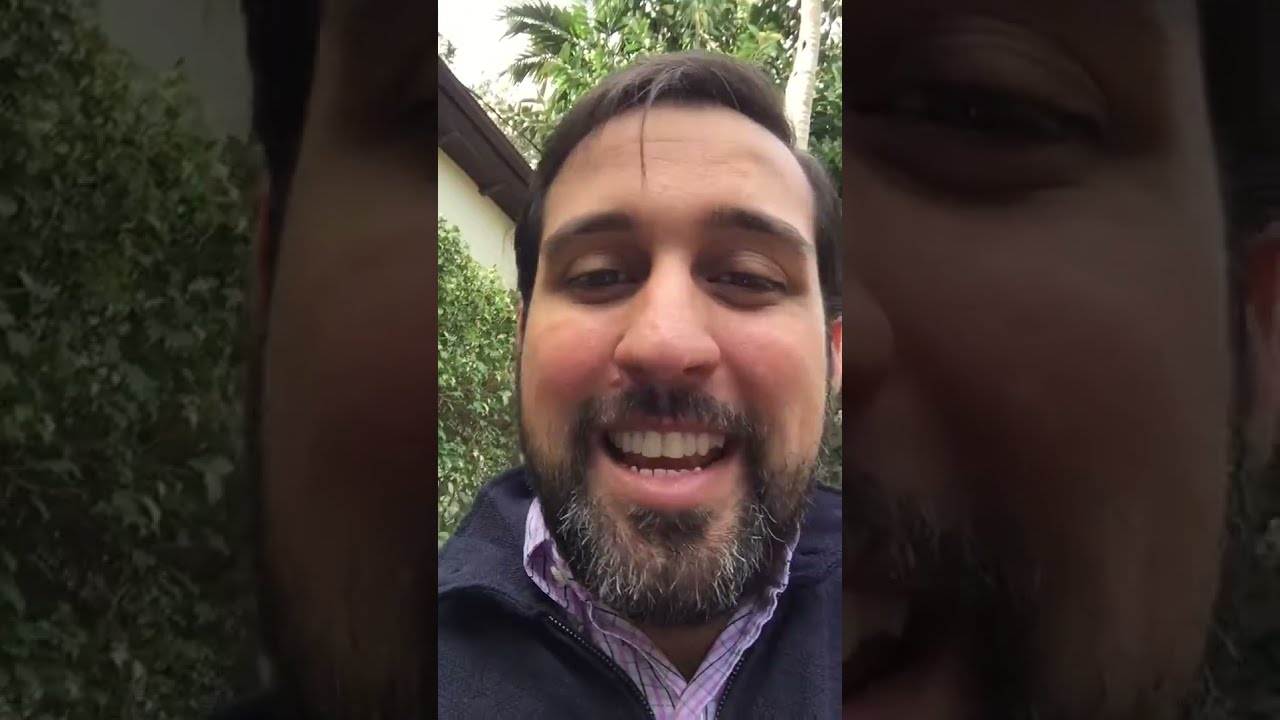This outdoor selfie captures a middle-aged man with brown hair, a full beard, and a mustache, seemingly in the middle of speaking. His mouth is open and his eyes have a distant gaze typical of someone engaged in conversation. He is wearing a navy blue sweater over a purplish dress shirt with collars, which has a plaid pattern. Behind him, the backdrop includes a cream-painted building with a wooden roof, as well as lush green foliage and trees. The man’s head is centered in the photo, with the trees framing both sides of him. The setting is clearly daytime, and the overall scene is bright and natural. The man has a pleasant expression and well-shaped face, making for a genial and engaging photograph.